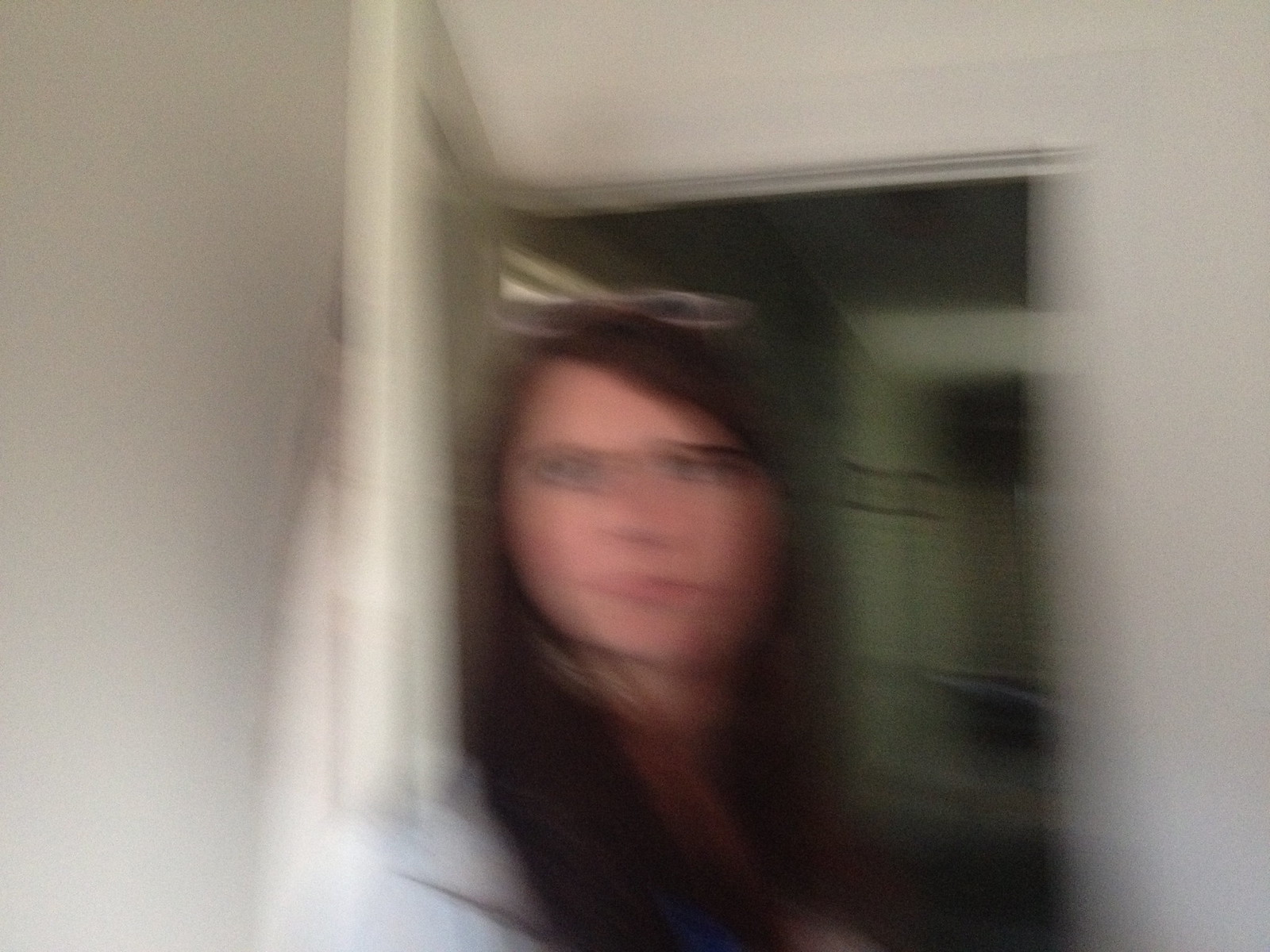The photograph is an extremely blurry indoor image featuring a Caucasian woman who appears to be in her late 30s or early 40s. She has straight, long brown hair, parted on the side, and wire-frame glasses perched on top of her head. She is wearing a white hoodie or long sleeve shirt. The setting shows her leaning through an open doorway with white walls and door frame. The background behind her is dimly lit, possibly illuminated by a distant light source or natural light, with some indistinct dark items visible. Her face, neck, and just the top of her upper body are vaguely discernible while the rest of her body remains out of the frame. The overall composition leaves the impression of her peering or leaning into another room, possibly through a door with an upper window, adding to the peculiar effect given the image's heavy blur.